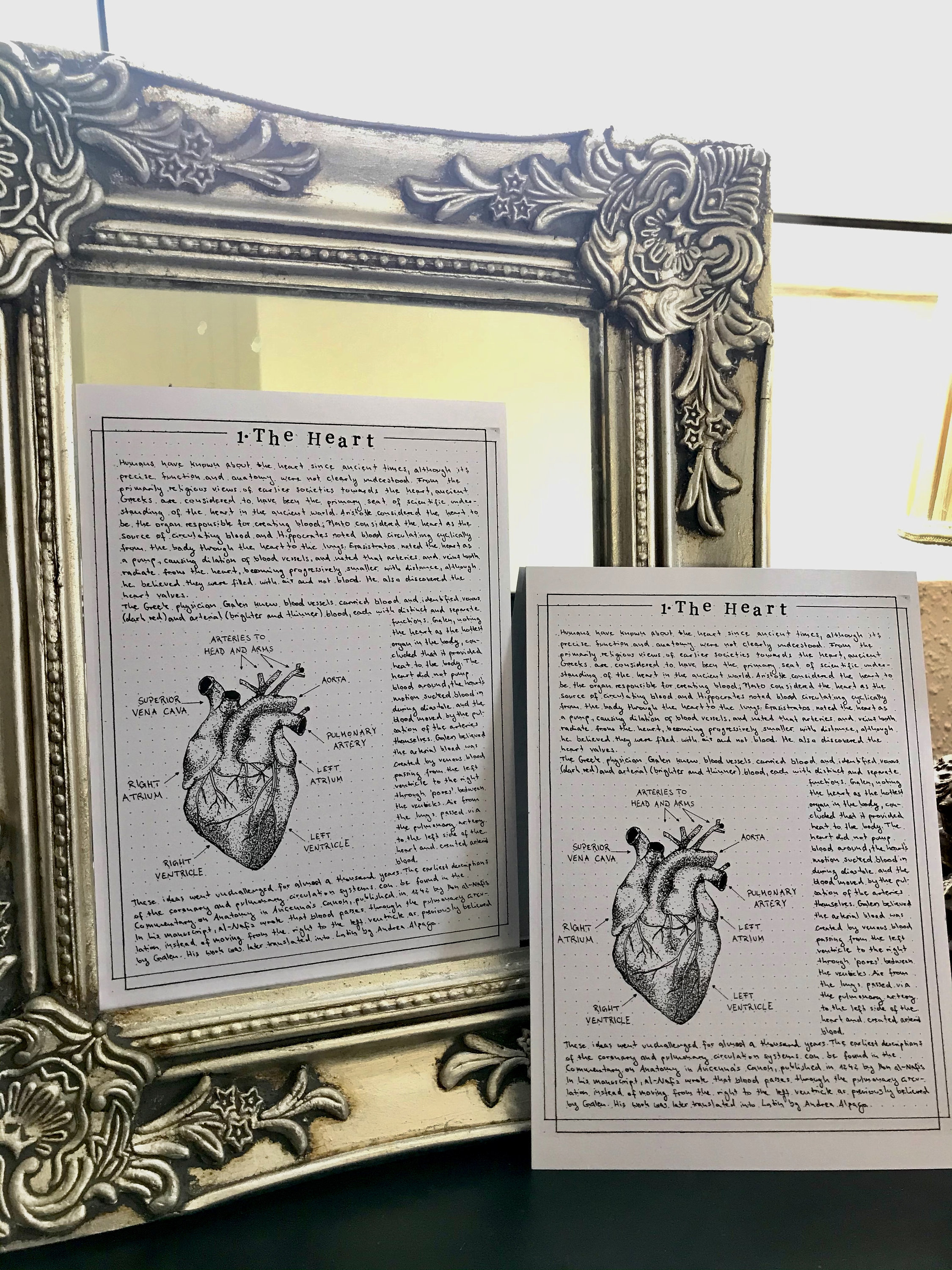This photograph captures two identical pieces of paper featuring a meticulously labeled anatomical diagram of the human heart. Both pages have a detailed illustration of the heart on the left side, with descriptions of various components such as the arteries, aorta, pulmonary artery, left atrium, left ventricle, right ventricle, right atrium, and superior vena cava. The right side of each page is filled with small, illegible text that extends downwards, ending with more text at the bottom. One of these pages is pressed against an ornate mirror with an elaborately designed frame, which appears metallic, potentially silver, with slight tarnishing and intricate floral patterns. The other page leans against the mirror to the side. The scene is set on a black surface, and in the background, a faint light is visible, adding depth to the composition.